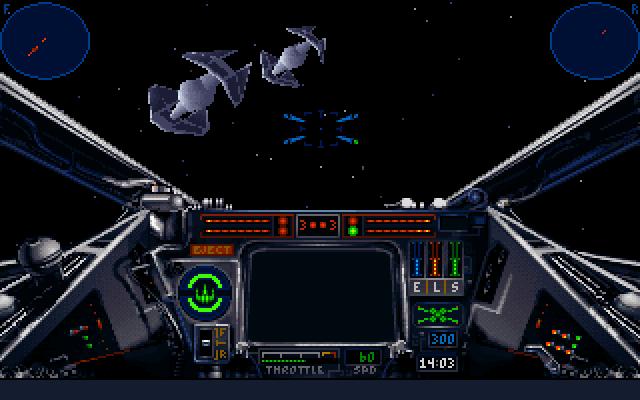The image depicts a view from the cockpit of a fighter jet within a 3D space-themed video game. The scene features a night sky with objects resembling satellites and Star Wars-style jet fighters engaging in combat in the background. Central to the image is a detailed control panel adorned with various buttons, dials, and lights in blue, orange, and green hues. Displayed prominently on the console are indicators for throttle, time, and speed, along with two round gauges located at the top left and right corners of the screen. The immersive setup suggests it could be part of an arcade or game room, or simply displayed on a computer screen.